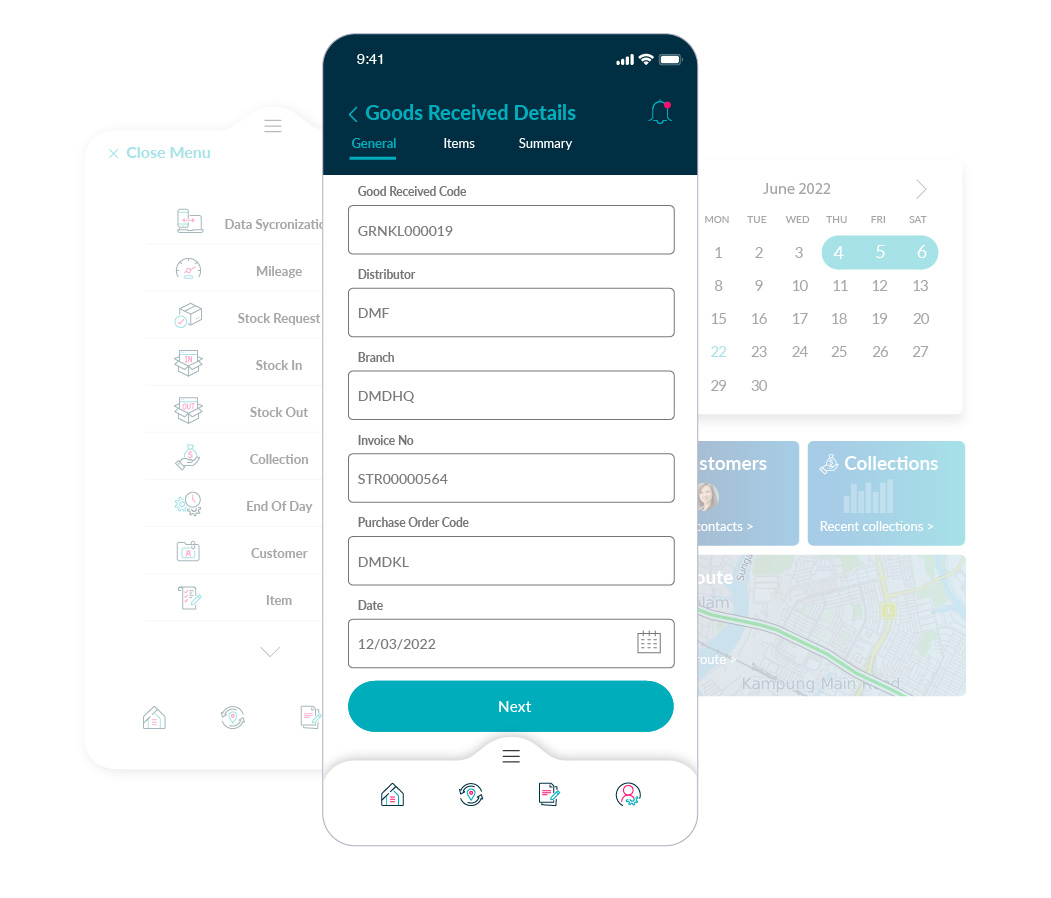The image displays a detailed view of two screens overlapping in a professional environment. The background screen predominantly features a user interface with several options listed: "Data Synchronization," "Mileage," "Stock Request," "Stock In," "Stock Out," "Collection," "End of Day," "Customer," and "Item." At the top-left corner, the option "Close Menu" is highlighted in teal. Additionally, a June 2022 calendar is visible on the right side, with the dates 4th, 5th, and 6th highlighted in teal.

In the foreground, another screen is displayed with precise information and status indicators. The top bar shows the time as 9:41, along with full battery and signal icons. Below that, a section titled "Goods Received Details" is highlighted in teal against a blue background. The "General" tab is active, indicated by an underline and a teal color. The screen lists several details including a "Good Received Code," distributor "DMF," branch "DMDHQ," an invoice number, a purchase order code, and the date "December 3, 2022." At the bottom, there is a prominent teal button labeled "Next."

Overall, the image captures a highly detailed snapshot of an organized digital workspace with layered information displayed prominently.